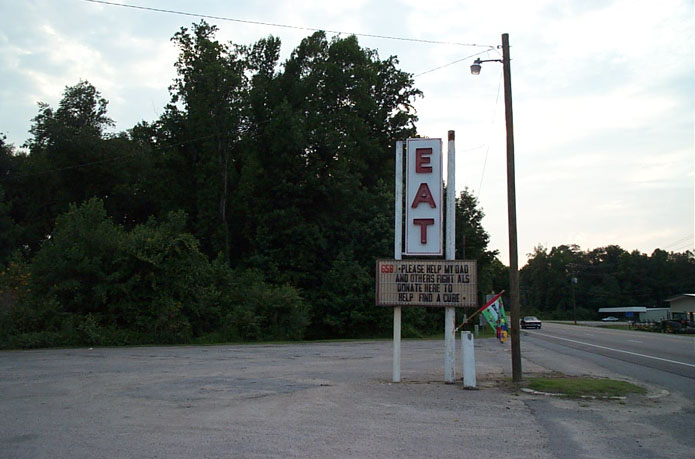In the foreground stands a retro diner sign, exuding a nostalgic charm with its bold red letters spelling "EAT" prominently against a white rectangular background. The sign is supported by sturdy white poles embedded into the concrete. Overhead, a streetlight is mounted on an electric pole situated slightly to the right of the sign, casting a soft glow over the scene. The backdrop features leafy trees, adding a touch of nature to the urban setting.

Adjacent to the iconic sign, a smaller changeable letter board implores passersby for support: "Please help my dad and others fight ALS. Donate here to help find a cure." The message is straightforward and heartfelt, appealing for aid in a personal battle against the disease. 

To the far right, an asphalt road stretches out with faint lane markings and a lone car driving off into the distance. Across the street, another building peeks into view, accompanied by an outbuilding and more flourishing trees, which add layers of depth and context to the scene. This picturesque setting blends elements of mid-century Americana and community spirit, capturing a slice of life where nostalgia meets earnestness.